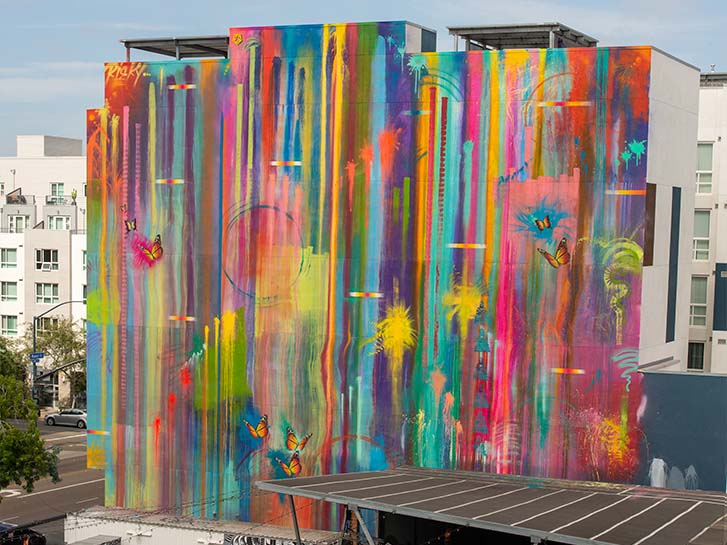The image showcases a tall building, vividly adorned with an extensive, vibrant graffiti mural that spans the entire visible wall. The mural presents an exuberant array of colors, resembling a rainbow, with shades ranging from red, orange, yellow, green, blue, light blue, and purple. Intricately painted monarch butterflies, with their iconic orange and black wings, embellish the wall, adding life to the colorful spectacle. The building, possibly multi-story with an unclear purpose, is situated in an outdoor, daylight setting under a clear blue sky. The surrounding buildings in the background are predominantly white or cream-colored, featuring glass windows and terraces, providing a stark contrast to the colorful mural. A single tree stands to the left of the mural, and portions of streets, including pavements, lampposts, and some parked cars, are visible. Notably, beneath the vibrant mural, a section of the roof appears to be fitted with solar panels. The entire scene captures a lively urban environment accentuated by the striking, multicolored graffiti art.